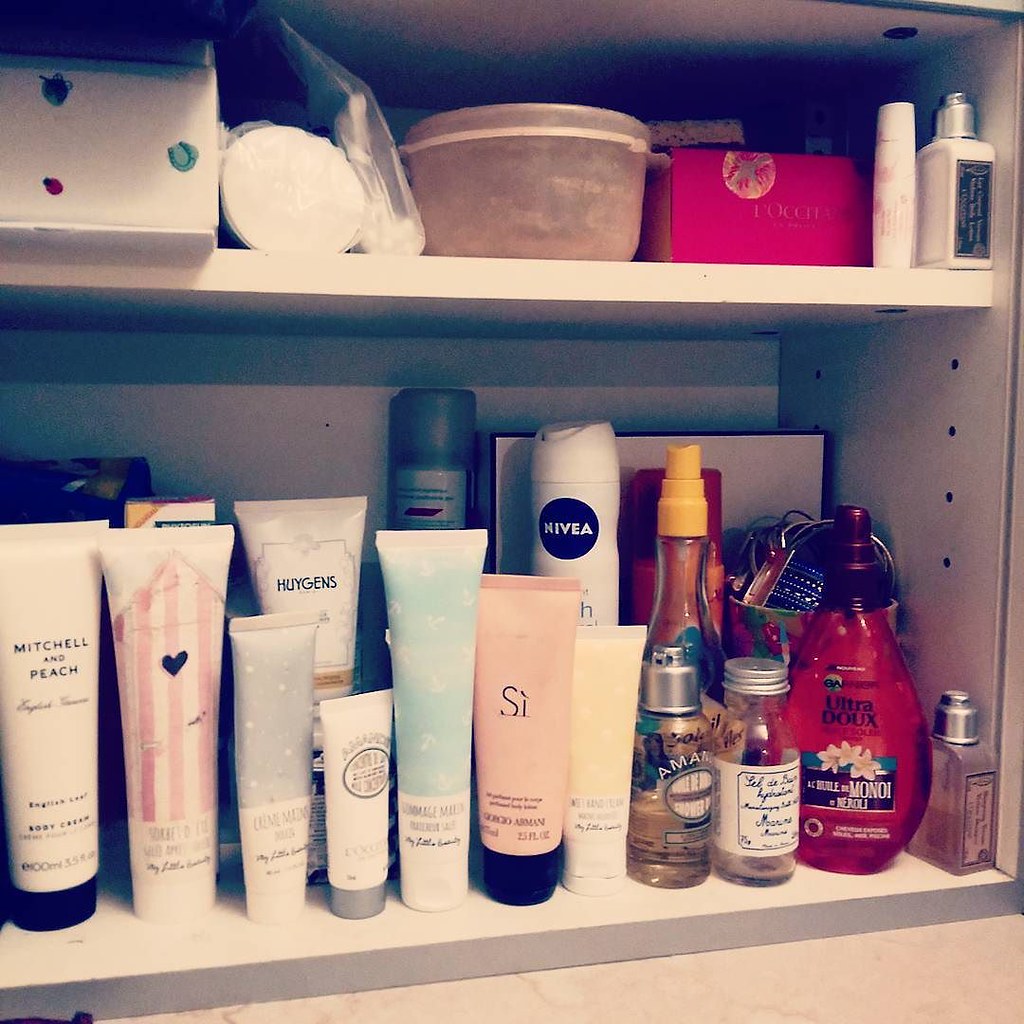This photograph captures the organized interior of a cabinet with two white shelves. The bottom shelf, larger in size, is systematically lined with an assortment of cosmetic products predominantly in vertical tubes, standing upright on their caps. From left to right, there is a white tube labeled "Mitchell and Peach" with smaller text reading "Body Cream." Next, a tube is adorned with pink and white stripes featuring a black heart design. Following this is a sleek silver tube and a white tube marked "Hugh Jens." Although some tube labels are difficult to decipher, a variety of other tubes, bottles, and spray bottles are visible. At the far end of the shelf, a perfume bottle stands out. The top shelf houses a shoe box and several other containers, adding to the array of stored items within the cabinet.